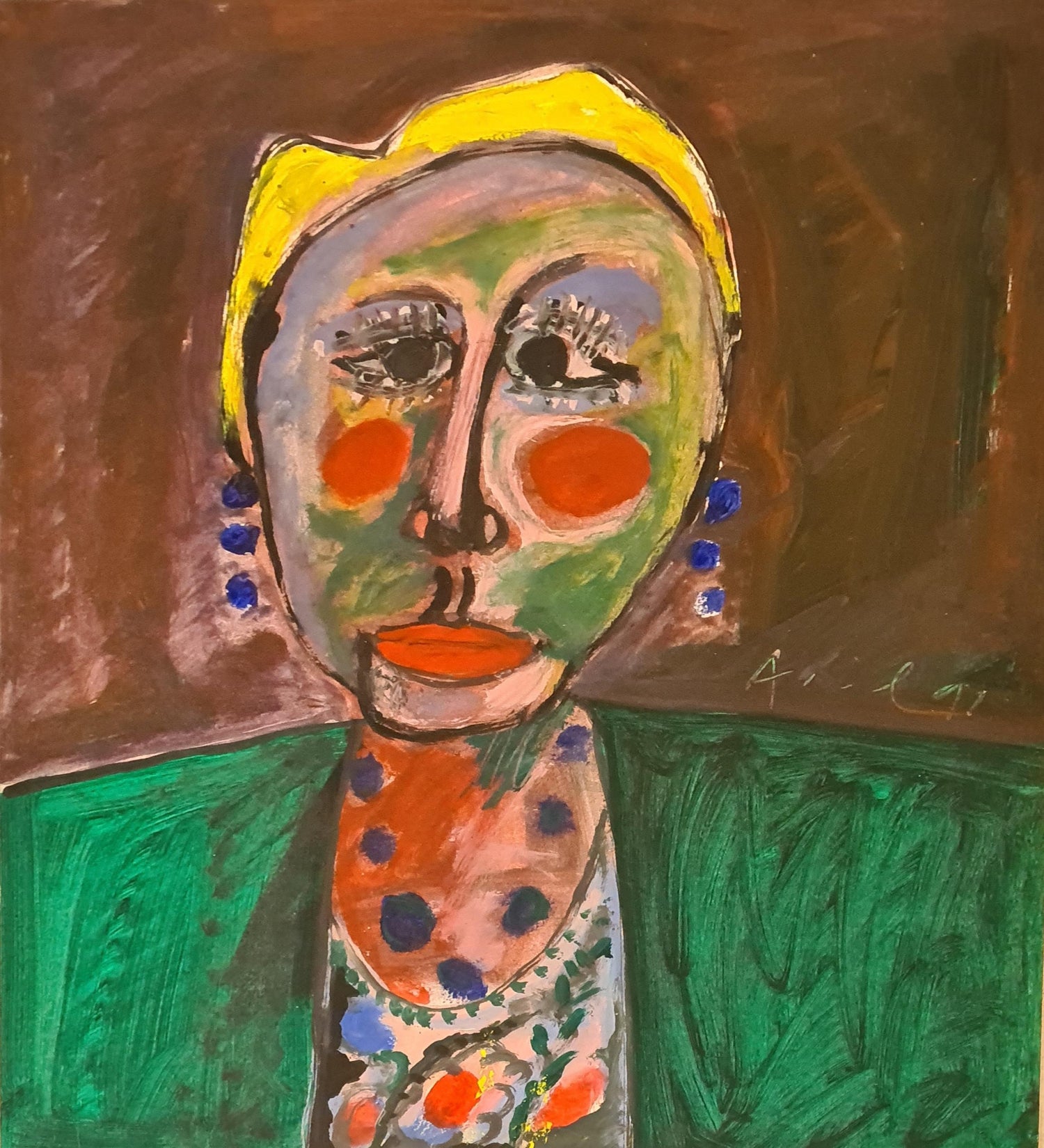This oil painting presents a strikingly abstract portrait of a woman set against a brown background. Her facial features are rendered with a blend of colors including green, purple, and red, giving her a vivid and somewhat surreal appearance reminiscent of Picasso's style. Her blonde hair contrasts with the green and yellow hues on her face, where her eyes, placed unnaturally close to her thin nose, have black centers that seem to pierce through the viewer. She dons a dark green sport coat over a flower-patterned shirt, adding to the eclectic mix of colors and textures that define her look. Small, blue beaded earrings dangle from her ears, matched by a similar necklace, reinforcing her vibrant yet abstract presentation. The painting's composition emphasizes bold geometric shapes and broad shoulders, with her head appearing disproportionately small. A barely legible signature in adult handwriting lies on the right side, suggesting the artist's intention to mimic a child's rendition, further enhancing the whimsical and unconventional essence of the piece.